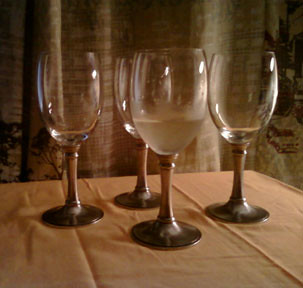This is a photograph of four wine glasses arranged closely together on a table covered with a sandy brown tablecloth that shows visible fold lines and slight lumps from the glasses being moved. The goblets are clear glass with dark-colored bases and stems, which exhibit shades varying from dark brown to bronze, possibly due to wear and use. Only the wine glass positioned closest to the viewer contains liquid, which is about one-third full with a slightly opaque, light-colored liquid that might be white wine, while the other glasses appear empty. Behind the table, there is a floral-patterned curtain that combines hues of brown and beige, adding a touch of vintage aesthetic to the scene.